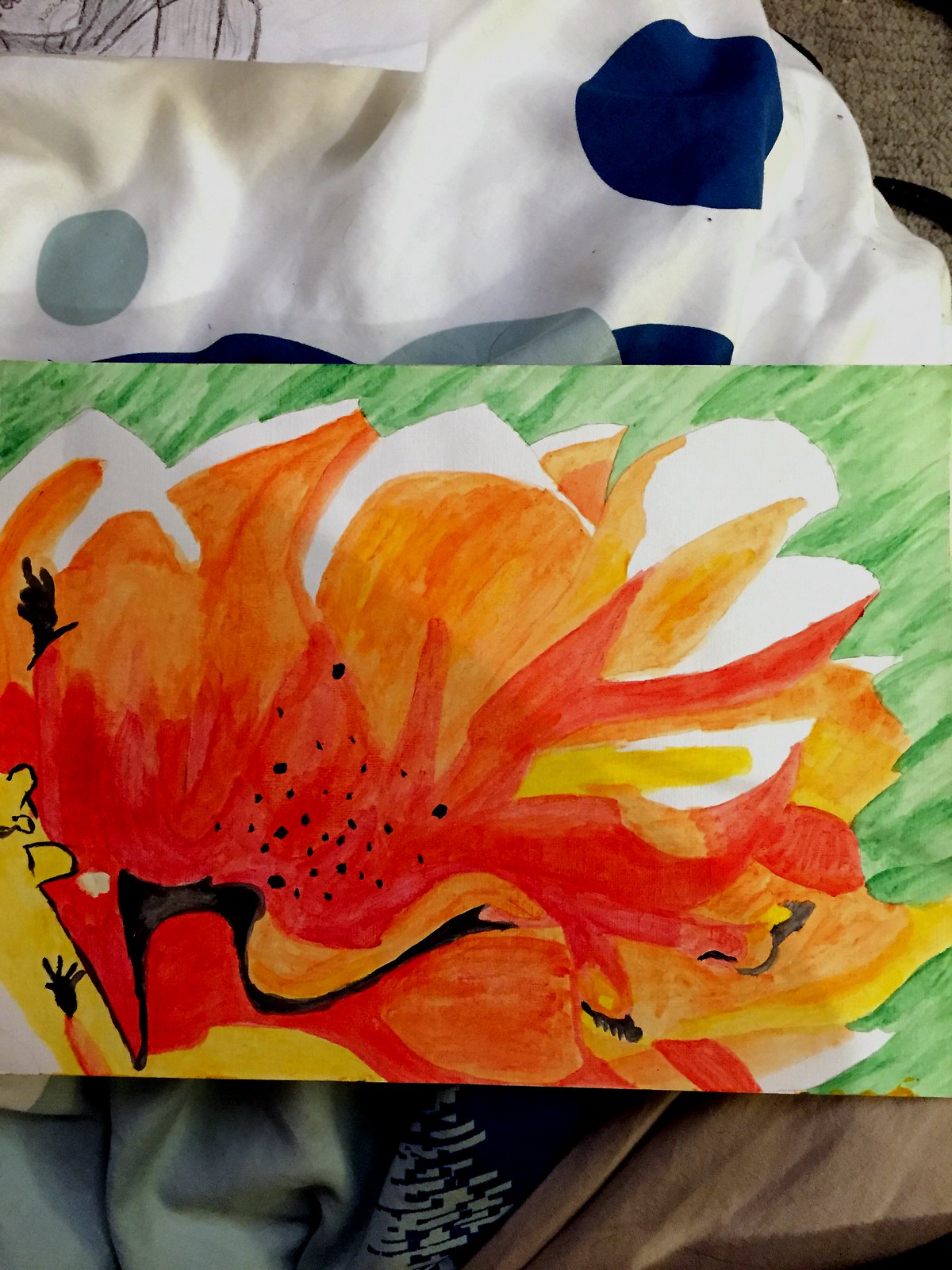This vibrant painting by an artist masterfully blends floral elements with subtle human features. The focal point of the artwork is an orange flower adorned with spots, transitioning gracefully from deep orange to yellow-orange, then melding into white. The backdrop is predominantly green, providing a striking contrast. At the bottom of the painting, the artist has intricately included parts of a human figure: an arm with a hand, discernible fingers, and suggestive contours of an eye, chin, brow, or nose. Curving black lines weave through these elements, enhancing the intricate details and adding a layer of depth. An eyelash is subtly depicted at the bottom center, while what seems to be a cactus or another hand appears at the top left. The painting is displayed against a textured fabric surface, possibly a sheet, tablecloth, pillowcase, or comforter, featuring a mix of stripes and dots. This exquisite composition captures a harmonious fusion of botanical and human forms, reflecting the artist's imaginative vision and thoughtful interpretation.